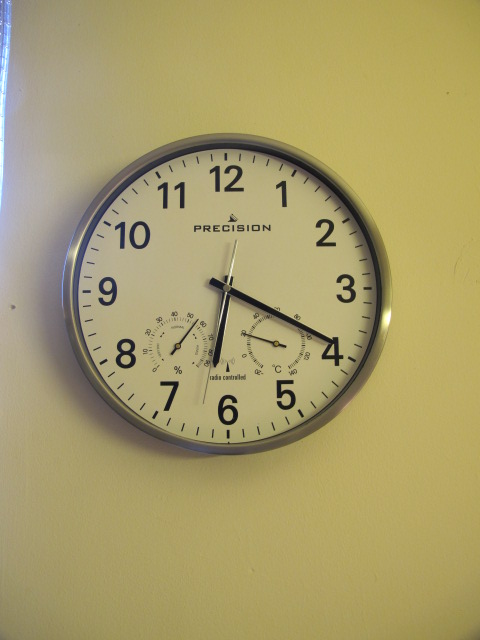In this detailed photograph, a wall-mounted circular analog clock is prominently featured. The clock has a pristine white face encased in a shiny, metallic silver border, followed by a black inner border. The black numerals, ranging from 1 to 12 with additional minute markings, are clearly visible on the face. Below the numeral 12, the brand name "Precision" is inscribed, while above the numeral 6, "Radio Control" is noted in small text. 

The clock displays the current time as 6:20 with its black hour and minute hands contrasted by a slim silver second hand. On the clock face, there are two additional dials: one on the bottom left indicating humidity with percentages from 0 to 100, and one on the bottom right showing temperature in degrees Celsius, ranging from -20 to 140. The wall behind the clock has a subtle greenish-gray tone, adding to the overall ambiance of the image. This multifunctional clock not only tells time but also provides humidity and temperature readings, making it both a practical and aesthetically pleasing object.